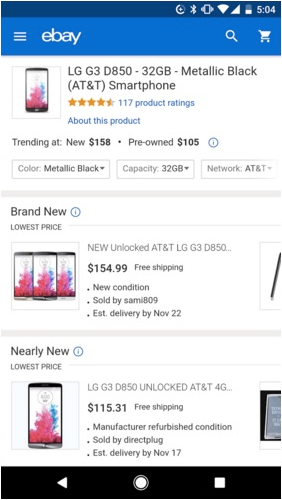This is a detailed screenshot from the eBay app, taken on a person's cell phone. At the top of the image, there's a dark blue banner displaying the eBay logo in lowercase white letters, accompanied by a search icon and a shopping cart icon. Below this, a photograph showcases an LG G3 D850 smartphone, described as a 32-gigabyte model in metallic black, compatible with AT&T.

The product has garnered a 4.5-star rating from 117 reviews. Additional information provided includes:
- Trending prices: New at $158, pre-owned at $105
- Color: Metallic black
- Capacity: 32 gigabytes
- Network: AT&T

Below the main information section, there are listings for different sales options:
1. A trio of smartphones identical to the one in the primary image:
   - Listing: New unlocked AT&T LG G3 D850
   - Price: $154.99 with free shipping
   - Condition: New
   - Sold by: SAMI 809
   - Estimated delivery: By November 22nd
  
2. Another sale option featuring the same smartphone:
   - Listing: LG G3 D850 unlocked AT&T 4G
   - Price: $115.31 with free shipping
   - Condition: Manufacturer refurbished
   - Sold by: Direct Plug
   - Estimated delivery: By November 17th

The image contains no people or animals.